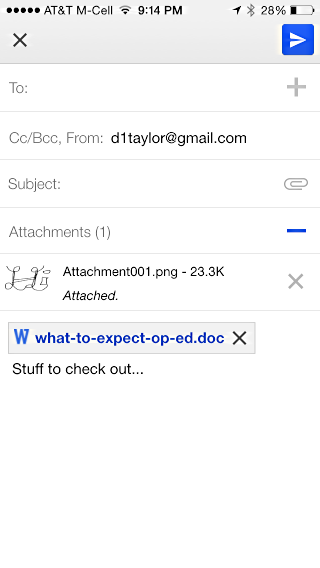A detailed caption for an image of an email on a phone screen:

The image shows a smartphone screen displaying an email interface. The top right corner of the screen indicates the battery life at 28%, while the time shown in the middle of the banner is 9:14 PM. On the top left, the phone carrier is identified as "AT&T" with five signal strength dots.

The email interface includes multiple sections. The "To" field, "Carbon Copy (CC)" field, and "Blind Carbon Copy (BCC)" field are  present but not filled out. The "From" section is filled out with the email address "d1taylor@gmail.com." The "Subject" field is empty, indicating no subject has been entered for this email. Below the subject field is an attachment field that displays an attached document. The attachment is titled "what to expect op-ed," is a Word document, and has a size of 23.3 KB. The body of the email simply reads "Stuff to check out below." The phone screen appears to be showing the Gmail app or another similar email client.